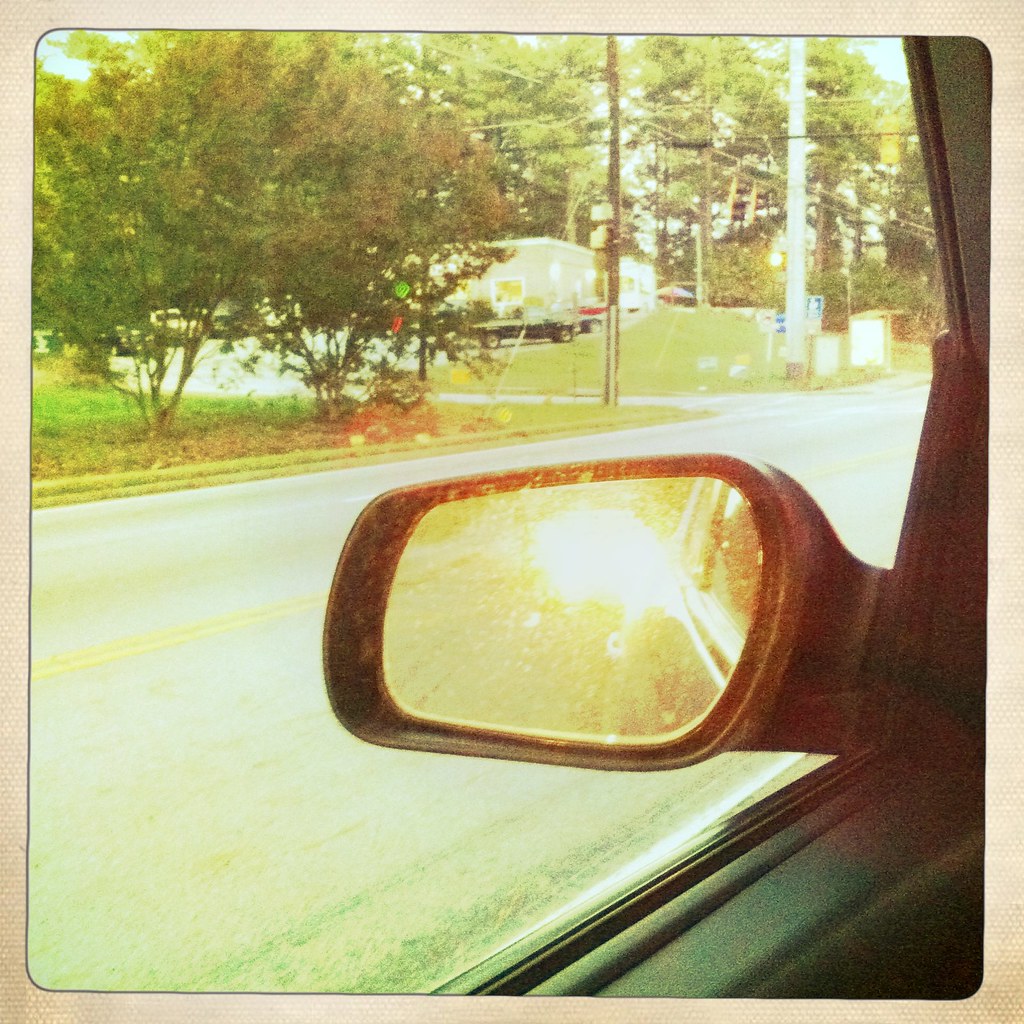The image captures a view from the driver's side window of a car, with the edge of the car door and side mirror prominently visible. A bright yellowish light reflects in the mirror, which also shows a glimpse of the car’s side. Visible through the window is a gray street with double yellow lines, leading to an intersection where a road branches off to the left. Trees, which are green and somewhat spindly, line the separated roadways. A grassy area stretches toward a building in the background, beside which several cars, including a dark-colored pickup truck, are parked. Two poles—one brown and another grayish and thicker—stand against the skyline, supporting various wires. Small, unreadable signs adorn the gray pole. The picture has a tan-colored border with rounded corners, mimicking the appearance of a photo set in an album. Inside the car, reflections of light create a red spot below a small green spot in the top middle of the image.